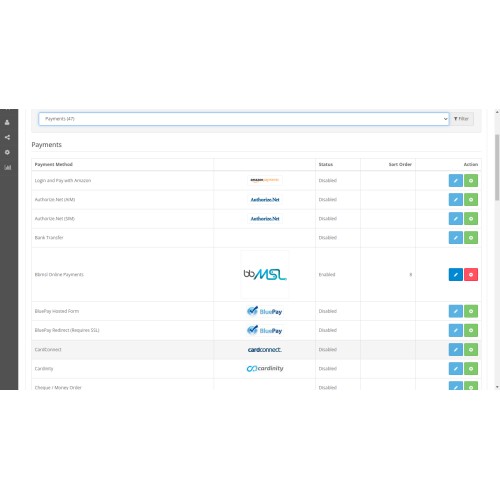The image depicts a low-resolution screenshot of a payment settings interface. The background is predominantly white or gray with a vertical black strip on the left side, containing icons for profile, share, a circle, and a graph. At the top of the page, there is a search bar and a drop-down menu, though the text is undecipherable. A button resides on the right side of this top row, but its label is also unclear.

The main content area prominently features headers labeled "Payments" and "Payment Method." Below "Payment Method," there are four listed items, although the specific details for each item are not readable. Adjacent to these payment methods, under the header "Actions," there are two buttons: one green, possibly indicating "proceed," and one blue with a pencil icon suggesting an edit function. In the center of the page, the text "BBMSL" is visible.